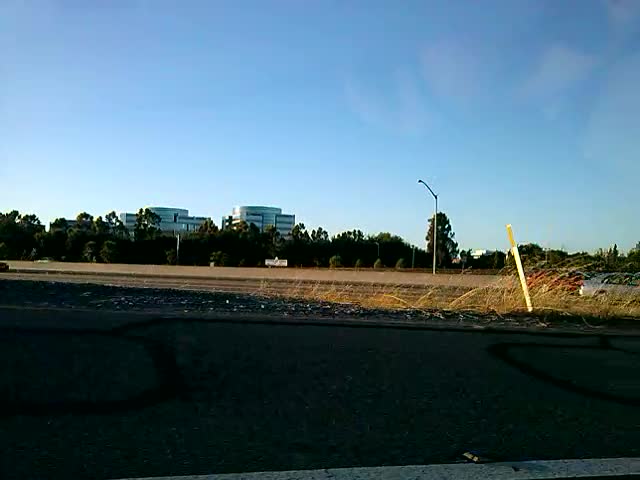The image captures a vibrant outdoor scene under a clear, blue sky stretching across the entire top of the frame. Central to the image is a lush tree line of verdant green foliage, behind which two tall buildings with distinct rounded tops made of concrete can be seen. In the foreground lies a dirt field, bordered by patches of dry grasses and a prominent white sign post. The very front of the image features a dark street, partially visible, with a white middle line marking on the left edge, cut off at the bottom. A tall light pole stands in the field across the street, adding vertical interest to the scene. To the right, a silver car is caught mid-motion, heading out of the frame beyond the dry grasses.